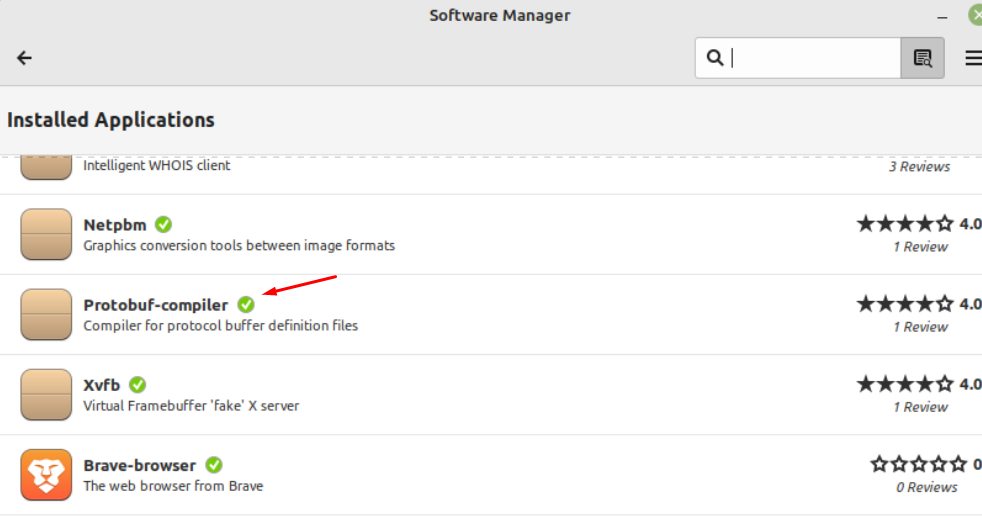The screenshot showcases the interface of a desktop screenshot application labeled "Screenshot". At the top-middle section of the application, the title "Software Manager" is prominently displayed against a grey background. To the lower right of this title, there's a search bar. On the extreme top-right corner, a cutoff green 'X' button is visible, alongside an icon of three black horizontal lines, likely representing the settings menu. Towards the left, a back button is presented as a left-facing black arrow.

Beneath these elements, a lighter grey background section contains the header "Install Applications." The list of applications begins with the "Intelligent Whois Client," which has three reviews. Following this is "NetPBM," which features a green checkmark and the description "Graphics Conversion Tools between image formats." This application boasts a rating of four out of five stars based on one review. Next is "Protobuf-Compiler," marked by a diagonal red arrow indicating its selection. Its description reads "Compiler for Protocol Buffer Definition Files," and it also holds a four-star rating from one review. Below, "XVFB" is listed, described as a "Virtual Frame Buffer Fake X Server" with a consistent four-star rating and one review. Finally, the "Brave Browser" is mentioned as the "web browser from Brave," currently showing zero stars due to a lack of reviews.